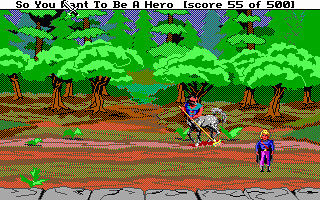In this vintage video game still, set in a pixelated, rudimentary environment, two characters occupy the scene. On the left, a centaur—a mythical half-man, half-horse creature—stands firmly on a patch of brown dirt. Adjacent to him, in the bottom-right corner, a heroic figure with blonde hair is dressed in striking purple tights and a cerulean blue cape. The backdrop is lush with many green trees, displaying detailed leaves and brown trunks, hinting at a forest setting. At the top of the image, black text poses the question "Do you want to be a hero?" Below this query, the current score is depicted as 55 out of a possible 500, suggesting an ongoing adventure or challenge.